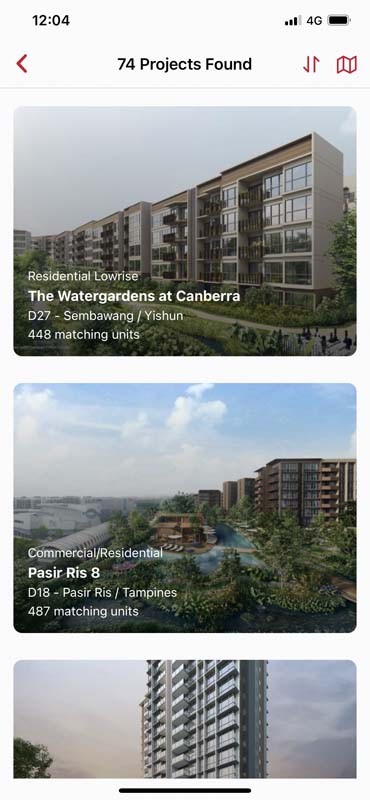Screenshot of a mobile device displaying several details. The time at the top reads 12:04, with a signal strength of three bars on a 4G network and an almost full battery icon. The interface shows a red back arrow on the left. The screen indicates in black text that there are "74 projects found." Two red icons are visible: one with vertical arrows and another resembling a map. The first image showcases a mock-up of a five-story residential low-rise complex named "The Water Gardens at Kanbara," featuring 448 matching units and surrounded by greenery. The second image presents a multi-story commercial-residential building with 487 matching units, surrounded by water and ample greenery.